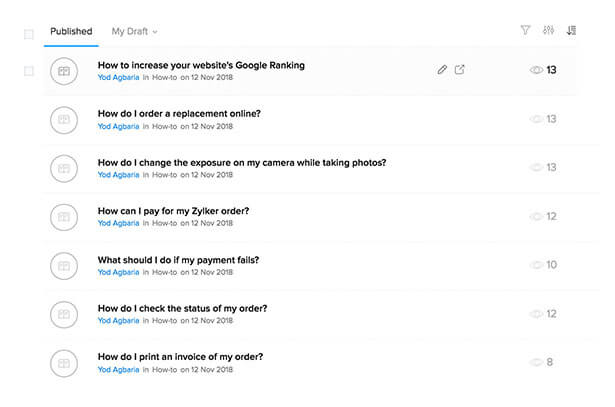This is a screenshot of an online content publishing panel set against a white background. At the top left, the word "Published" stands out in bold black letters, accentuated by a blue line underneath. Just to the right, "My Draft" appears in bold gray letters. Below, a vertical list of published how-to blogs is displayed. 

The first blog entry is titled "How to Increase Your Website's Google Ranking," with the author's name in bold font appearing underneath, accompanied by the category "in How-to" and the publication date "12th November 2018." Adjacent to it on the right are an edit button and a share button. On the far right, an eye icon indicates that the post has been viewed 13 times.

Continuing down the list, the second entry is titled "How Do I Order a Replacement Online?" This entry is by the same author and was published in the same category and on the same date—12th November 2018. Similar to the first, it shows an eye icon on the far right indicating 13 views.